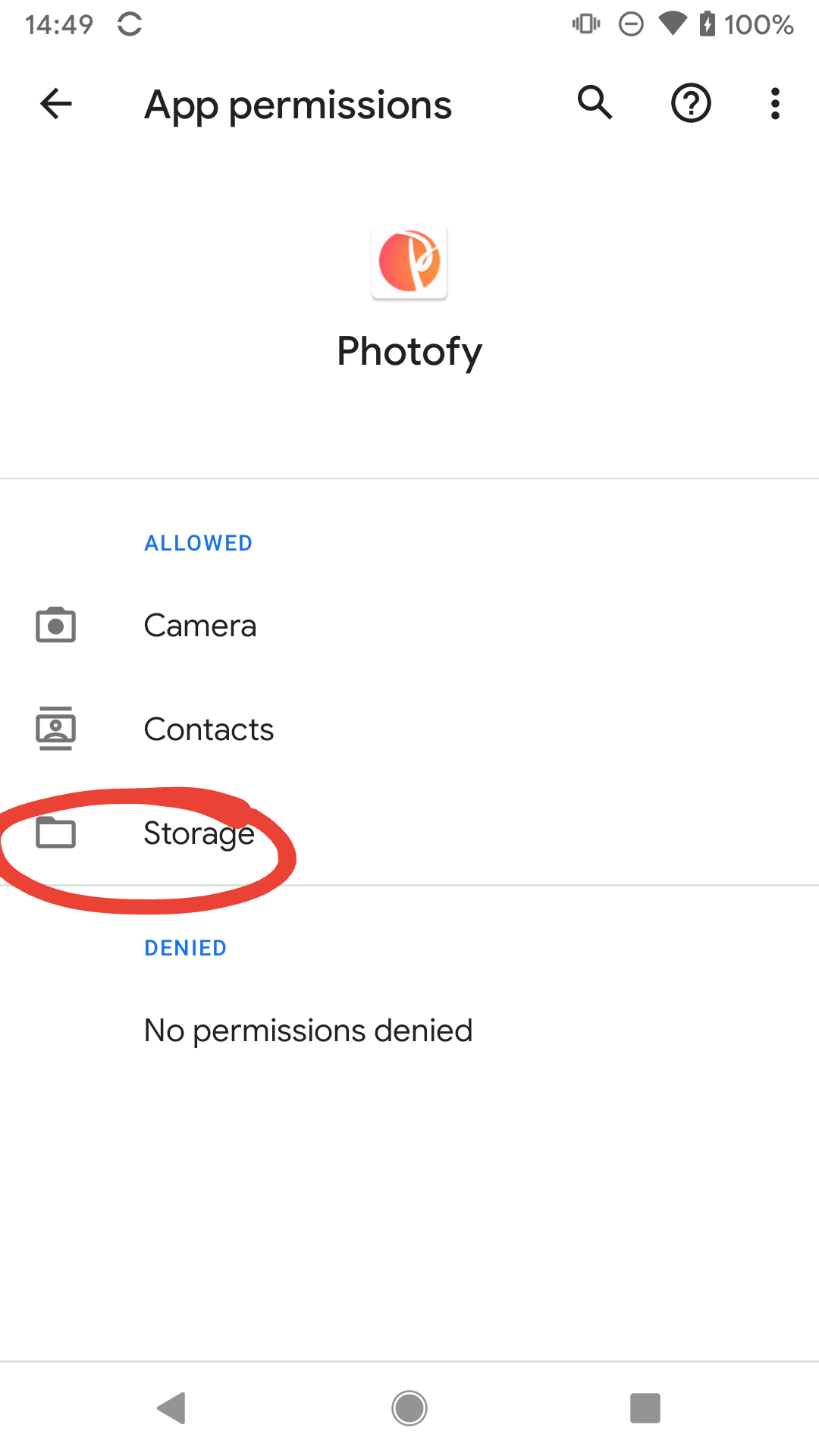This screenshot captures the "App Permissions" page for the mobile application "Photofy." At the top of the screen, the status bar displays the current time (14:49) on the left, and icons for a fully charged battery and vibrate mode on the right. 

Just below the status bar is the title "App Permissions," accompanied by a magnifying glass icon, a question mark icon, and a vertical ellipsis (three dots) for additional options on the far right. 

The "Photofy" app is highlighted, with its distinctive logo—a cursive "P" inside an orange circle—positioned above the app name. 

The permissions are categorized into two sections: "Allowed" and "Denied," both text headers shown in blue. 

- Under "Allowed," circled in red, are three permissions accompanied by icons:
  - Camera (camera icon)
  - Contacts (contacts icon)
  - Storage (folder icon)

- Under "Denied," the text reads "No permissions denied."

The footer of the screen includes three navigation icons: a triangle pointing left, a circle in the center, and a square on the right.